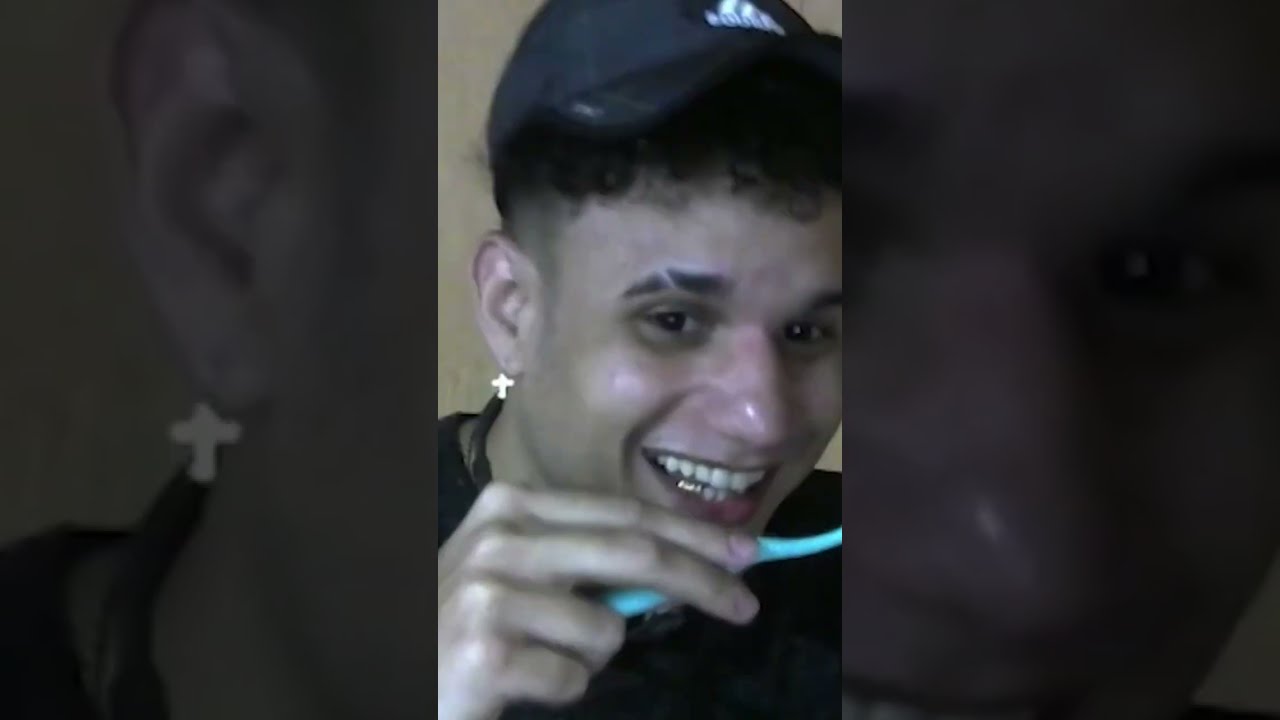The image is a creative, horizontally rectangular photo montage of a young, dark-haired man wearing a black Adidas baseball cap with white lettering and a black shirt. His right ear sports a silver cross earring. In the main, central image, the young man's face is turned slightly left, with his brown eyes looking to the right. He has a distinct slash through his right eyebrow. He's smiling softly with his mouth slightly open and is holding a turquoise blue object, possibly a toothbrush, between his thumb, pointer, and middle fingers, while his other fingers are curved down.

Behind him, a large, close-up of his face forms the background, blending more darkly into the overall composition. Adjacent to the central image, the montage is divided into three vertically rectangular sections that feature different parts of the same main image. On the left, you can see the back of his head, emphasizing his curly hair. On the right, a clearer view of his face highlights his calm and engaging expression.